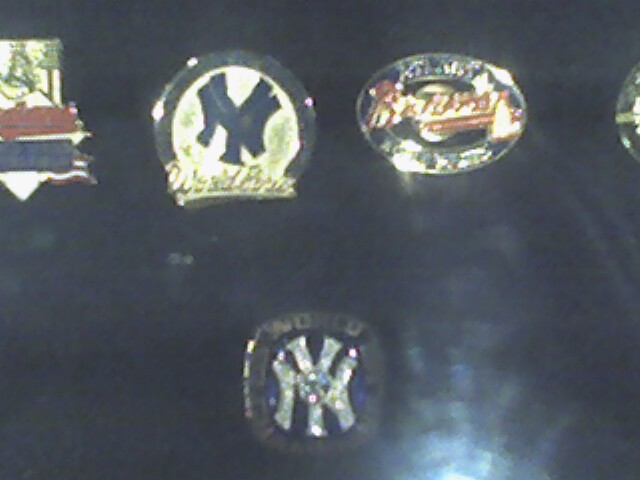The photograph depicts a collection of four sports-themed pins or rings, although the image is very blurry and poorly lit. The background is solid black with a slight flash visible in the lower right. On the lower part of the photo, there is a New York Yankees pin or ring with a golden border and a blue center featuring an intertwined 'N' and 'Y' with a diamond where the letters intersect. It appears to bear the word "World Series" around the edges, though the text is difficult to read.

Above this, there are three more pins or rings. The top middle pin is circular with a slight blue border and almost identical 'NY' logo, accompanied by the word "World" and another partially legible word that might start with 'B'. On the top left, there's a dark-colored rounded square pin with the 'NY' logo, encircled by a dark blue border with some illegible gold script beneath it. The top right pin is oval-shaped, likely featuring the Braves logo in red script and bordered in silver, although the exact details are obscured due to the poor quality of the photograph.